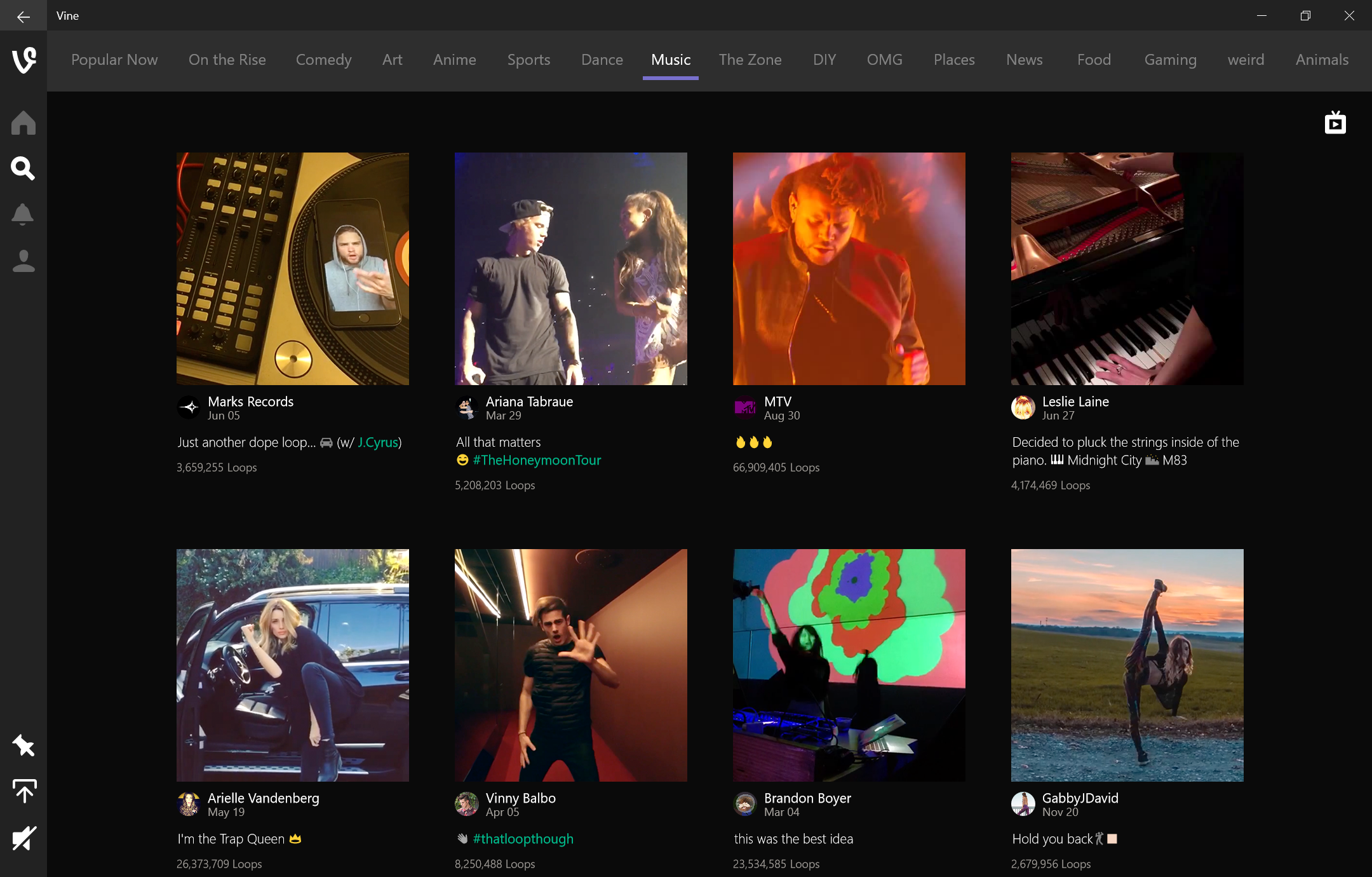This image is a screenshot showcasing the interface of the Vine app. The Vine logo, which features a stylized capital letter "V" with a curly extension on the right side, is visible. Down the left side of the screen, there are four navigation icons representing the home page, search function, notifications, and personal profile, depicted as a silhouette of a person.

At the top of the screen, there are several clickable categories: "Popular Now," "On the Rise," "Comedy," followed by a variety of other genres including "Art," "Anime," "Sports," "Dance," "Music," "The Zone," "DIY," "OMG," "Places," "News," "Food," "Gaming," "Weird," and "Animals." The "Music" category is currently selected, highlighted with a brighter white text and a blue underline.

In the main content area, there are two rows of user profiles, each row containing four profiles. In the top row, the featured users are Mark's Records, Ariana Tambre, MTV, and Leslie Lane. The bottom row includes Arielle Vandenberg, Vinny Balbo, Brandon Boyer, and Gabby J. David.